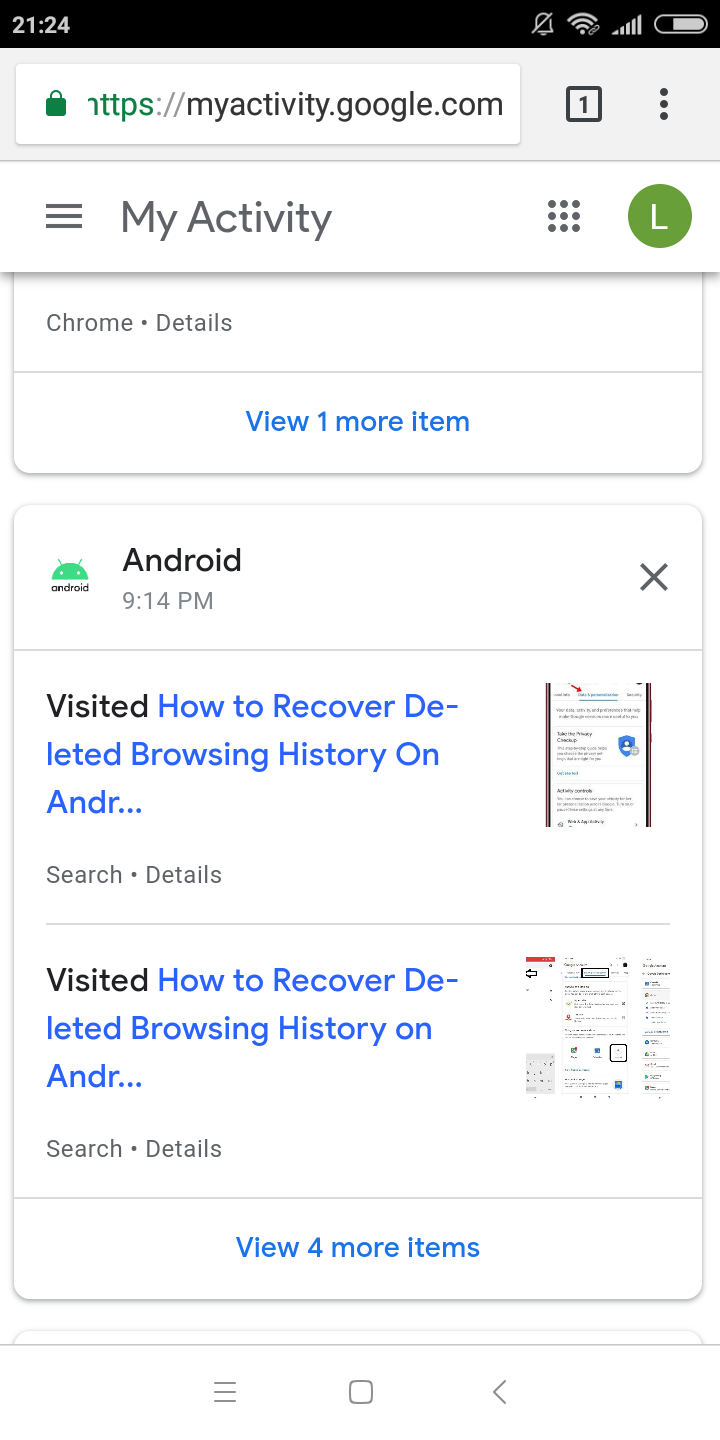The image displays a user interface with various elements. At the top, there's a black status bar. On the left side of this bar, "21:24" is displayed, indicating the time. Adjacent to the time, icons show a full Wi-Fi signal, full cellular signal bars, and a battery icon indicating about 25% charge. There are three horizontally stacked lines (a menu icon) also present on the bar. On the right side, the text "My Activity" is prominently displayed.

Below the status bar, the interface consists of multiple sections. The top section displays three rows of three dots each and features a green circle with an "L" in the center. Underneath this, there is a box labeled "Chrome details" with a blue hyperlink reading "View one more item" below it.

Further down the interface, the text "Android 9:14 PM" is shown with an "X" mark to the right and a light grey line beneath it. Below the line, the word "Visited" is in black, followed by a blue hyperlink that reads "How to recover deleted browsing history on Android, search details." This phrase appears twice in succession, each time with the tag "Visited" and a corresponding blue hyperlink.

Next to each hyperlink, there's an indistinct thumbnail image that is too small to identify. Finally, at the bottom of the interface, there is a blue hyperlink that reads "View four more items."